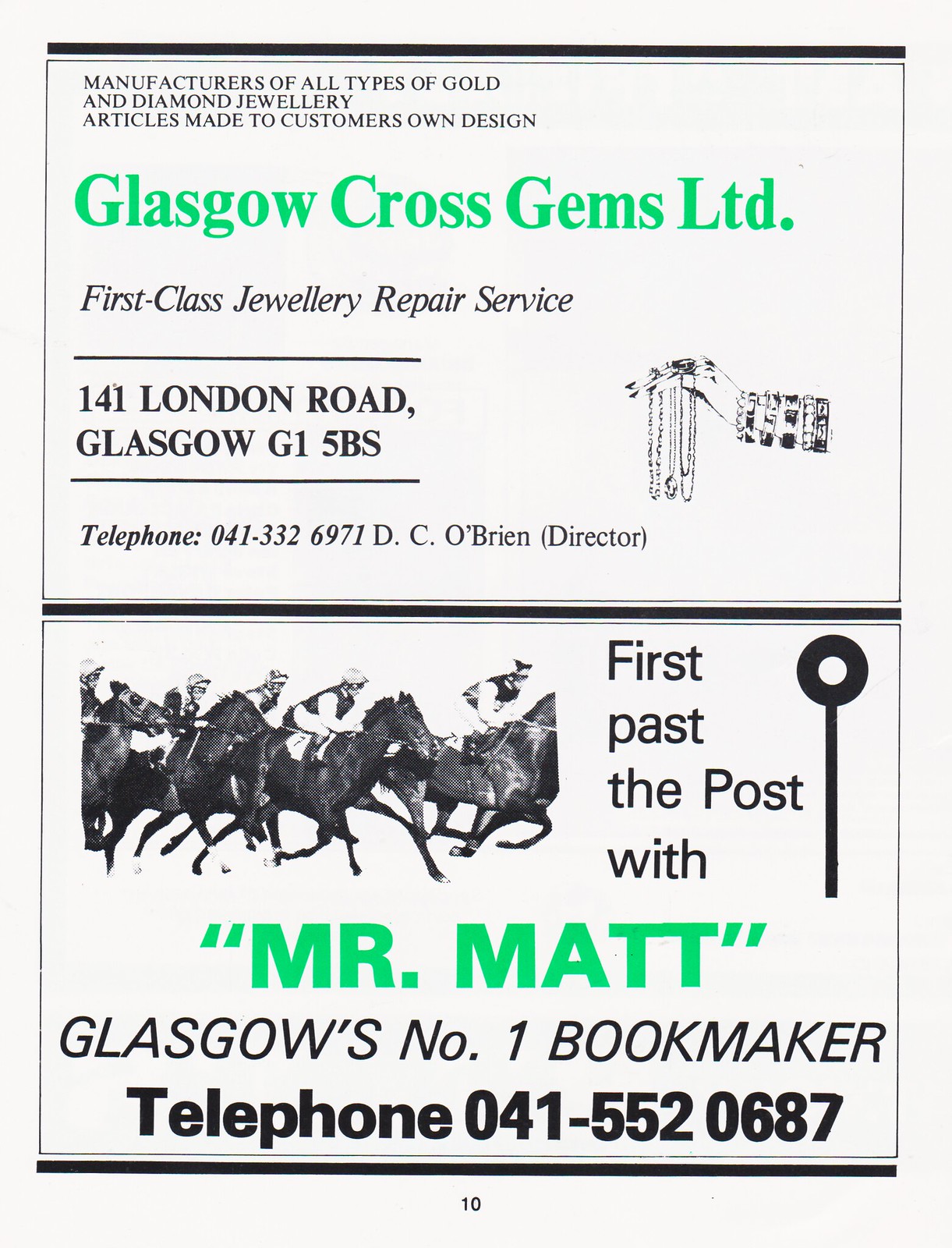The image appears to be a vertically-oriented advertisement from a magazine, with a light blue background and the page labeled as number 10. The page is divided into two sections, both featuring advertisements. The top section promotes "Glasgow Cross Gems Limited" with green lettering at the top, stating "Manufacturers of all types of gold and diamond jewelry, articles made to customers' own design." Below that, it reads "First Class Jewelry Repair Service, 141 London Road, Glasgow, G15BS," followed by the contact number "041-332-6971" and "DC O’Brien, Director." An illustration shows a jeweled hand adorned with numerous bracelets, rings, and necklaces, emphasizing the array of jewelry services offered.

In the lower section, the advertisement shifts focus to "First Past the Post with Mr. Matt, Glasgow's number one bookmaker." This section contains a group of jockeys riding horses, conveying the bookmaker theme. The contact number "041-552-0687" is also provided. Most of the text in the advertisement is dark, with the name of the place being advertised in light green, creating a distinct visual hierarchy in the layout.